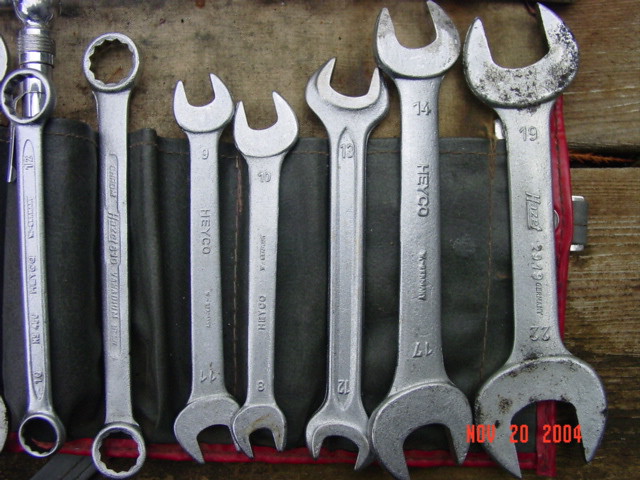This detailed close-up image, horizontally aligned, showcases several different sizes of wrenches laid out on an older wooden table or counter. The larger wrenches are positioned on the right side and decrease in size as you move to the left. Notable sizes visible on the wrenches include 19, 14, 13, 10, and 9, with the wrenches being either gray or silver in color. The two wrenches on the far left feature completely round ends, ideal for loosening bolts. Some wrenches are branded with "HEYCO," a known manufacturer. The image was captured on November 4th, 2020, as indicated by the red date stamp at the lower right corner. The wrenches are laid out on what appears to be a plastic mat that has red sewn edges, providing contrast against the wooden surface beneath.